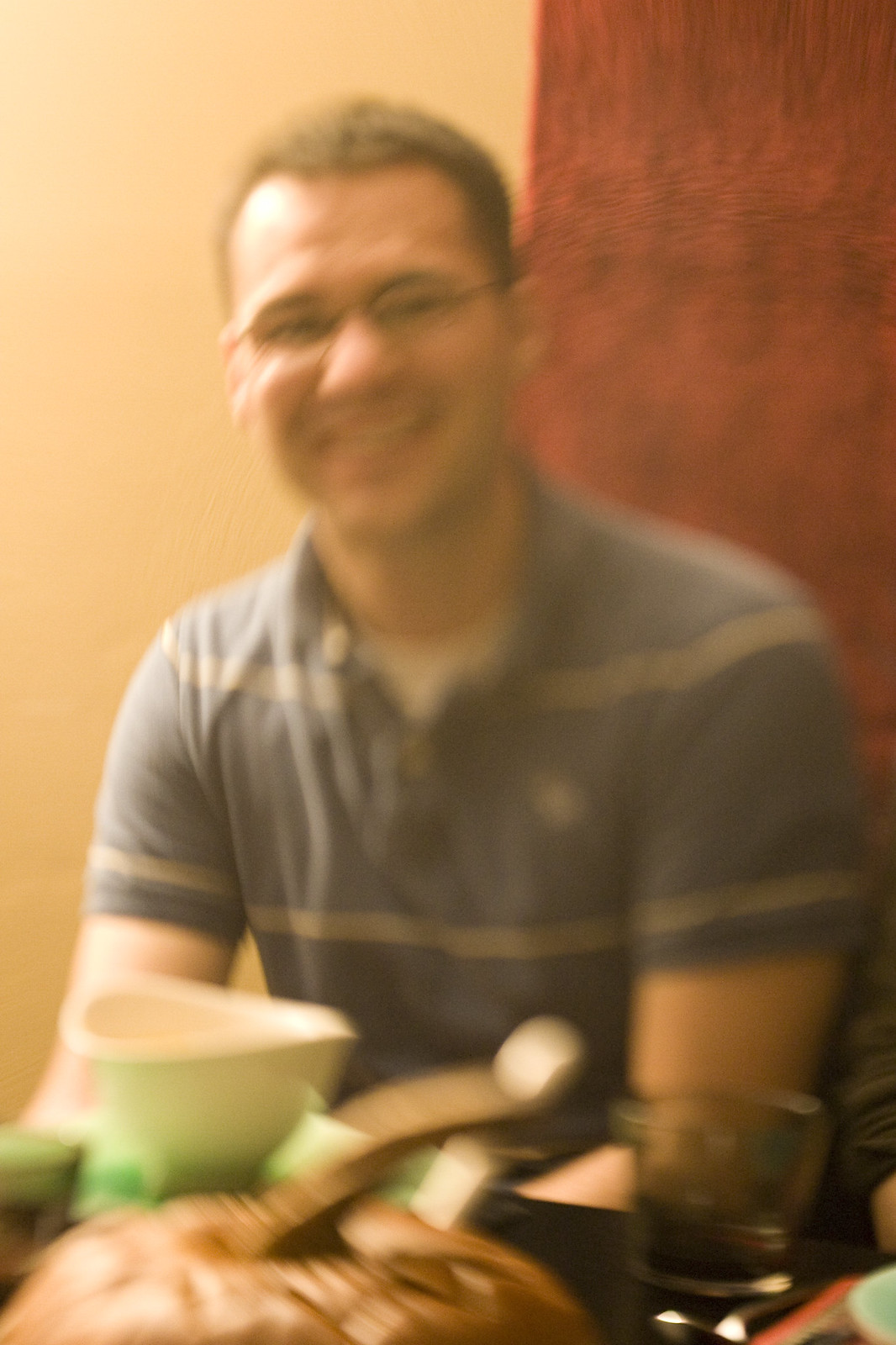A blurred image captures a moment of a man enjoying what appears to be a meal seated at a table. The backdrop features a two-tone wall, with the left side painted beige and the right a rusty brownish-red, adding a warm ambiance to the scene. The man, who is Caucasian, smiles warmly at the camera through his typical rectangular metal-framed glasses. He has short brown hair and is dressed casually in a white t-shirt beneath a collared blue polo shirt adorned with white racing stripes. In front of him on the table sits a white saucer, accompanied by a decorative pumpkin suggesting a Thanksgiving setting. To the side, a whiskey glass containing a small amount of whiskey hints at a relaxed and convivial atmosphere.